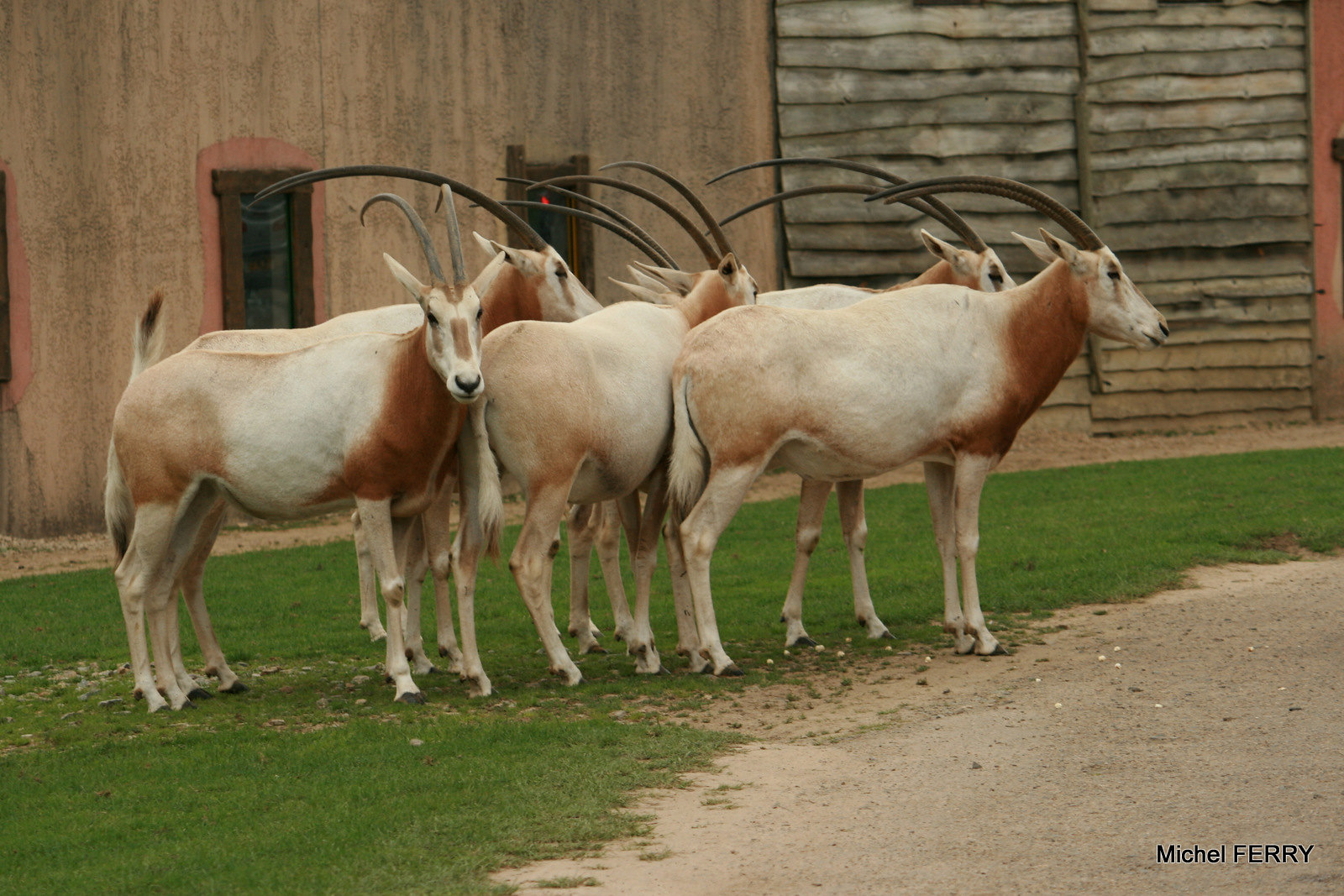In this detailed photograph, we see a closely grouped cluster of five goats standing on short, dark green grass by the side of a dirt road. These goats, varying in color from light brown to white, possess strikingly long, curved black horns that are at least a foot in length. Their necks and chests are primarily brown, their midsections and legs are white, and their rumps exhibit light brown patches. The goats' pointy ears and strong, long legs add to their robust appearance. 

In the bottom right-hand corner, the name "Michael Ferry" is subtly inscribed in small black text. The background reveals a rustic and decaying building made of brown stone with dark wood elements and some patches of black. This building, which features a pink stone-bordered doorway and another opening that might be a window, appears worn out and historic. In addition, there's a series of stacked brown firewood to the building's right-hand side. 

While most of the goats face away, seemingly interested in something happening down the road, one goat at the back turns to gaze directly at the camera, creating a sense of engagement with the viewer. This well-composed scene not only captures the steadfast nature of the goats but also provides a glimpse into a weathered, rural setting.